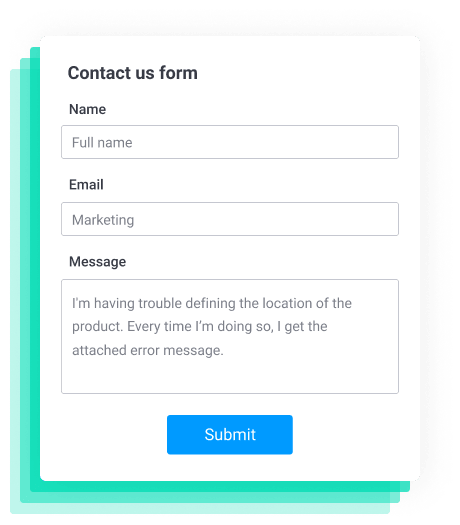The image showcases a "Contact Us" form pane prominently positioned on the screen. This form consists of a small white text box that encapsulates several user input fields. At the top, there's a text field labeled for entering the user's name, although it currently remains blank. Directly below, a slightly smaller field is marked for the user's email address, which is filled in with "marketing." Further down, a larger text area is designated for the user's message. The message currently displayed reads: "I'm having trouble defining the location of the product. Every time I'm doing so I get the attached error message."

At the bottom of the form, a blue "Submit" button stands out, highlighted and ready for selection. Below this primary contact form, the interface reveals a series of horizontal, gradient green tabs, indicative of multiple open tabs or sections beneath the current view. The overall screenshot displays only this form and these green tabs, obscuring other details such as the user's actual name or email address beyond "marketing."